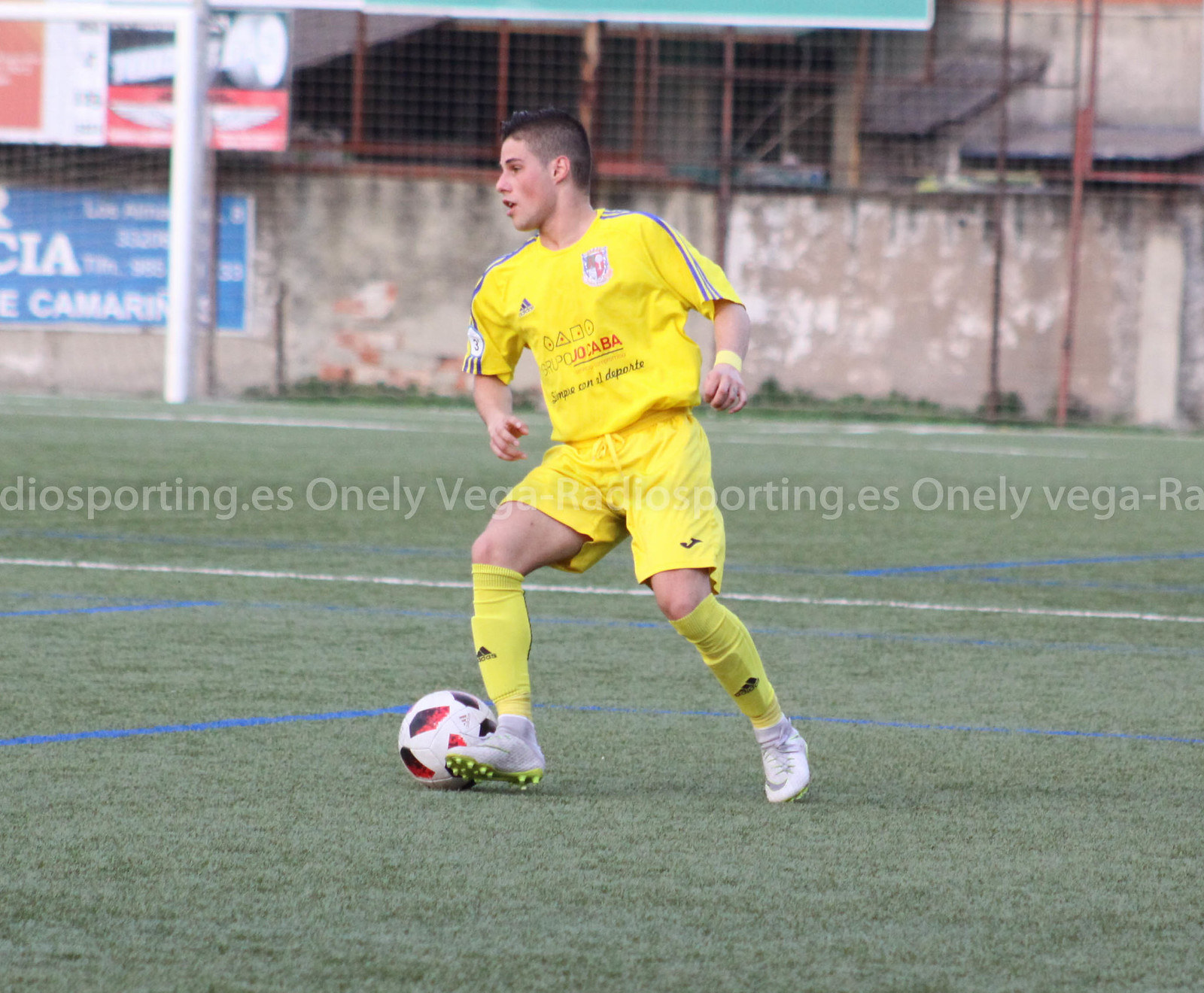The image captures a young soccer player, likely in his late teens to early twenties, skillfully manipulating a white soccer ball adorned with red and black blotches using the outside of his right foot. He is dressed entirely in yellow, sporting a uniform consisting of a yellow jersey with black and white stripes along the sleeves, yellow shorts, knee-high yellow socks displaying the Adidas logo, and white cleats with yellow soles. Additionally, he wears a yellow wristband. The soccer field is marked with white and blue lines, and in the background stands an aged barricade wall topped with a rusted cage-like structure. Billboards can also be seen in the background, while semi-transparent text reading "onelyvegaradiosporting.es" overlays the center of the photograph.